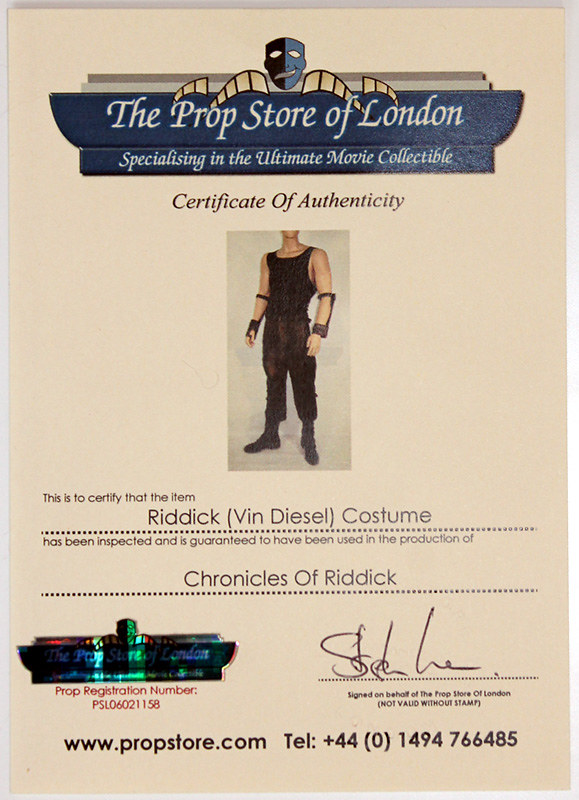The image is a vertically aligned rectangular certificate set against a light brown background. At the top, there's a blue header with a theatre mask icon and white text stating, "The Prop Store of London," followed by, "specializing in the ultimate movie collectible," in a smaller font. Below this, in black text, it reads, "Certificate of Authenticity." Beneath this section, there is a rectangular photograph of a man dressed in a black tank top, black arm bands, black pants, and black boots, although his face is not visible. Below the image, black text certifies that the item, a "Riddick (Vin Diesel) costume," has been inspected and guaranteed to have been used in the production of "Chronicles of Riddick." The lower left corner displays a prop registration number, and to the right, there's an illegible signature. At the very bottom of the certificate, the website "www.propstore.com" is listed alongside a telephone number.